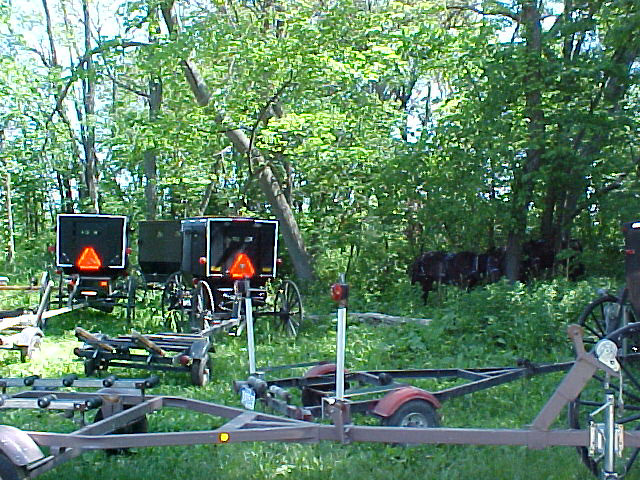This daytime outdoor photograph captures a serene, wooded scene teeming with life and objects. In the foreground, a pair of single-axle, brown metal trailers with two wheels and hitches sit amidst overgrown, wild green grass. The trailers have vertical parts with reflector lights on the back. One trailer faces directly right, while another angles slightly backward toward the right. Behind these trailers, partially obscured by the lush greenery, stand three black Amish-style buggies characterized by their large, round wheels and bright orange, triangle-shaped safety reflectors on their backs. Near these buggies and shaded by the dense, tall trees, are four large brown horses. A large, downed gray tree lies near the buggies, adding to the rustic atmosphere. The sky is light, potentially overcast, providing a soft light that brightens the rich greenery of the thick forest. The scene is tranquil, evoking the simplicity and quiet beauty of rural life.